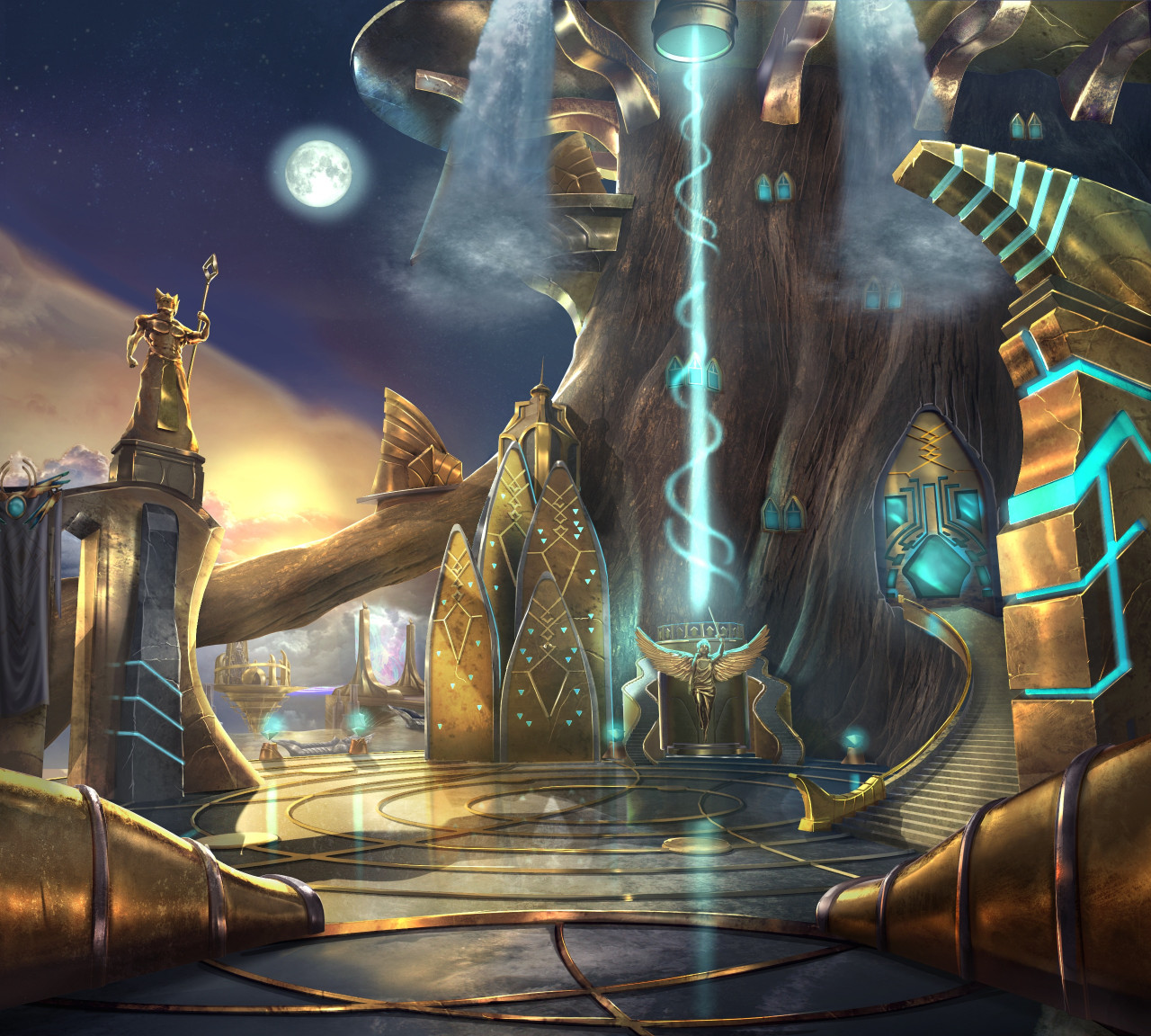A stunning CGI image, possibly from a video game or created through AI, depicts a celestial, regal scene filled with golden and teal hues. Central to the composition is a majestic golden figure that resembles an angel, holding a sword aloft as light beams down from a cylindrical device above, illuminating its form. To the left, there is another golden statue of a muscular man adorned with a crown, gripping a staff with a diamond-shaped head, seemingly gazing towards the moon in the top left corner, or perhaps the sun situated lower in the sky, demarcating the boundary between night and day at an angle. The scene is adorned with intricate golden inlays and circular patterns on a darker, marble-like floor. Supernatural elements abound, including swirling blue and teal lights, veins running through structures, and a prominent golden staircase curving towards a radiant blue doorway. The backdrop features a massive tree intertwined with metallic elements, enhancing the scene's enchanting, futuristic ambiance, reminiscent of an otherworldly realm or a space-age interpretation of Greek mythology.